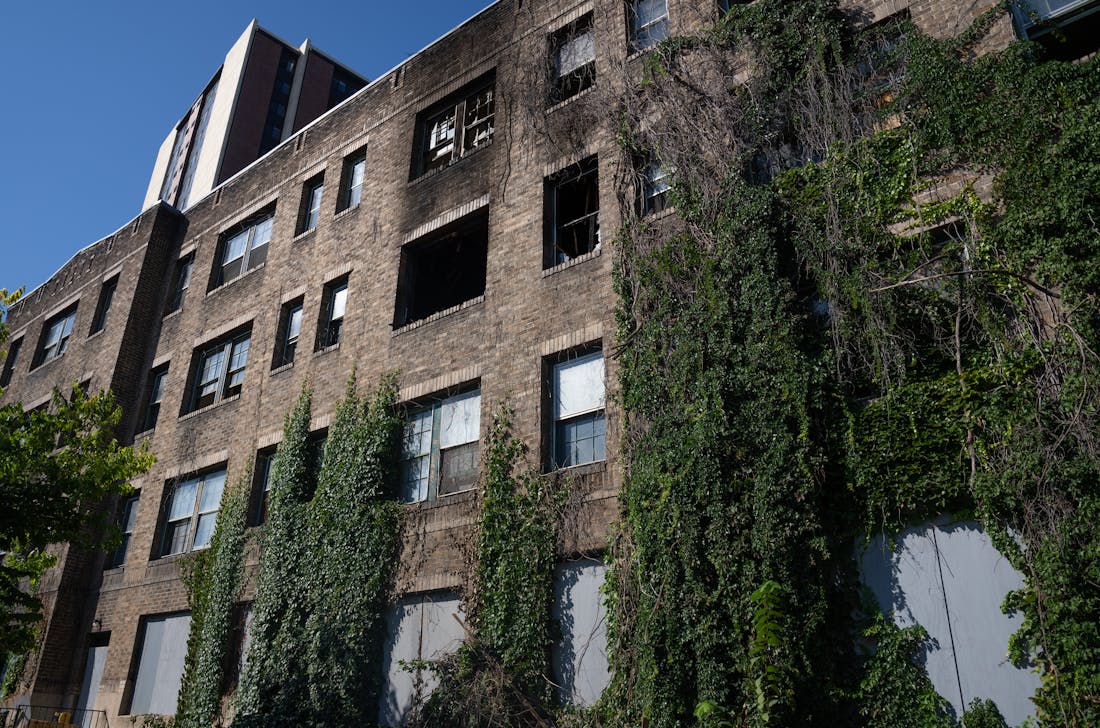The photograph captures the exterior of a towering, four-story abandoned building made of brown and gray bricks that appear weathered and charred in places. The facade is interspersed with large windows, many of which are either broken, missing, or covered by white surfaces or curtains, contributing to the structure's decrepit appearance. Dense green vines and some dead, brown vines snake up the sides of the building, further emphasizing its state of neglect and decay. On the left side, a singular tree stands amidst this scene of urban desolation. Above, a vivid, cloudless blue sky contrasts starkly with the sad, deteriorating edifice, creating a sense of abandonment and melancholy. At the upper left corner of the image, an obscured, possibly modern structure can be vaguely seen, its clarity diminished, adding another layer of ambiguity and contrast to the overall composition.